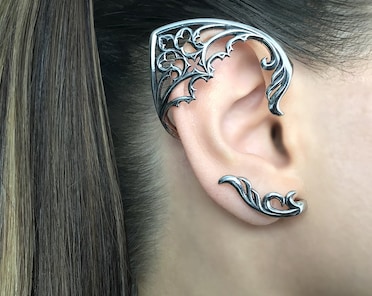This detailed rectangular photograph, approximately two to three inches wide and one and a half inches tall, captures the side profile of a Caucasian female's right ear and surrounding area. Her brown hair, highlighted and pulled up, drapes down the left side of the image, exposing her ear, a hint of her cheek, and part of her neck. The focal point is the elaborate metal ear cuff she wears, crafted from silver-colored metal. The intricate design wraps around her ear, from the top down to the earlobe, mimicking an elvish aesthetic with a pointed top that accentuates the ear. The adornment's pattern blends elements reminiscent of Victorian era designs, including hollowed centers and shapes that resemble crosses or flowers. Additionally, the cuff features a delicate fleur-de-lis motif with undulating lines below, and near the earlobe, a design that resembles a vine with three leaves, the bottom two curling gracefully like the letters C and S.